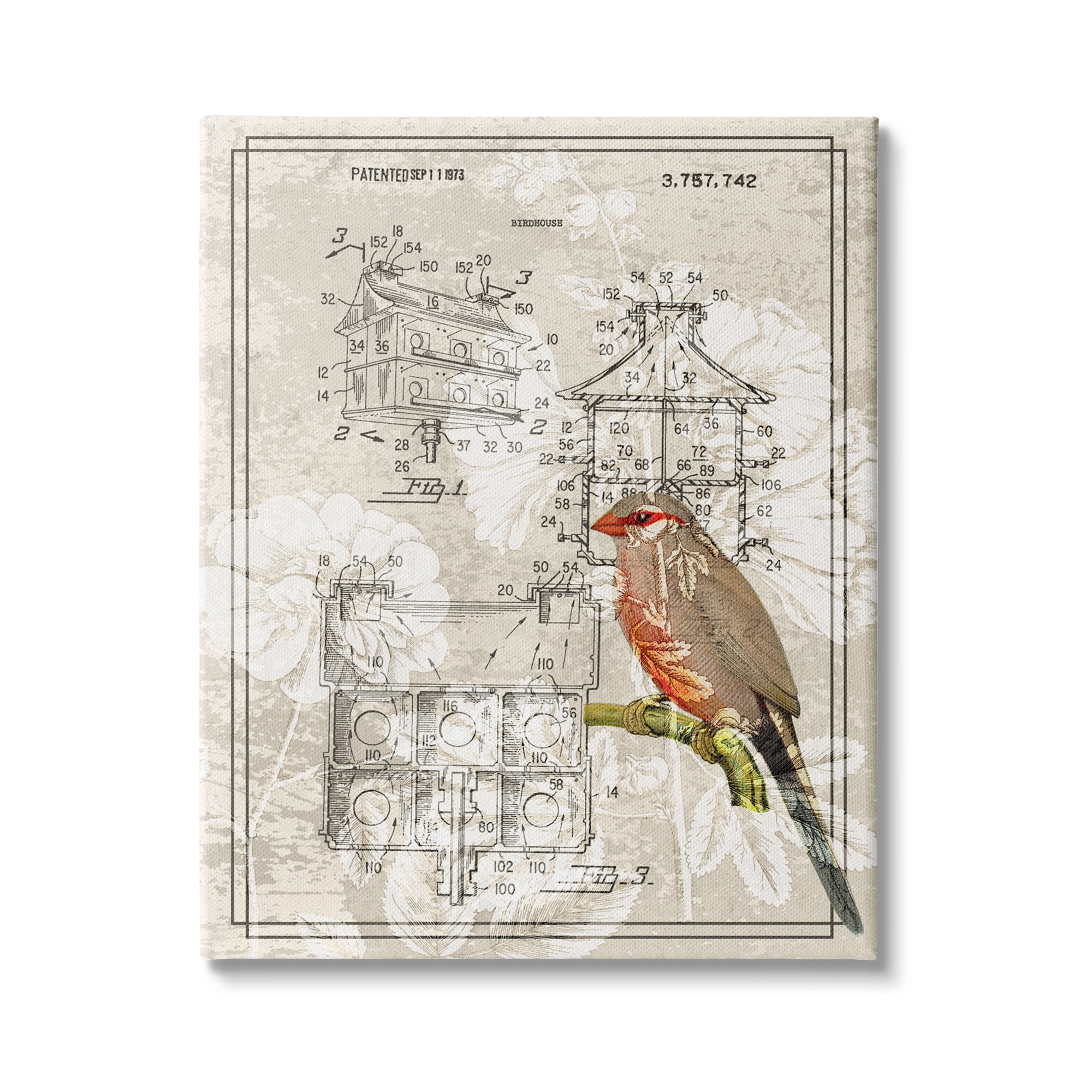This image is a detailed, patent-design diagram from September 11, 1973, featuring instructions on how to build a birdhouse. The background of the image has a creamy, light tan color adorned with white flowers, creating a decorative floral printed paper. A bird, possibly a cardinal, is perched on a green branch; this bird has distinctive red markings on its beak, eyes, and underbelly, with an overall light brown-gray coloration. The diagram, which includes multiple sketches of black-and-white birdhouse designs, shows detailed steps and components required for assembly, marked by numbers and arrows. The primary diagram features a square base with six smaller squares containing circles, while the second is a house structure with a triangular roof and various numbered parts. There is also a gray and white watermark running across the entire image.